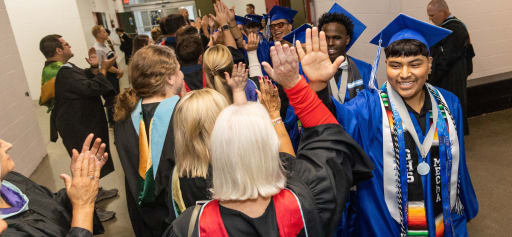In the photograph, a vibrant scene unfolds in what appears to be a school hallway, marked by gray hard flooring and white-painted cinder block walls. The hallway is filled with joyous energy as rows of individuals bask in the celebration of graduation. The right side of the hallway features a line of young graduates, most likely high schoolers, proudly donning blue graduation gowns and caps, adorned with white and blue tassels. One standout graduate also wears a white ribbon attached to a blue pendant and a sash that reads "GHS." These blue-clad graduates, predominantly men, are energetically high-fiving a line of individuals on the left side, who are wearing black gowns. This line includes older individuals, possibly teachers, administrators, or family members, who are eagerly engaging in the celebratory gesture, contributing to the heartening display of mutual encouragement and happiness. The atmosphere is electric, with smiles and raised hands filling the space, creating a palpable sense of achievement and community.